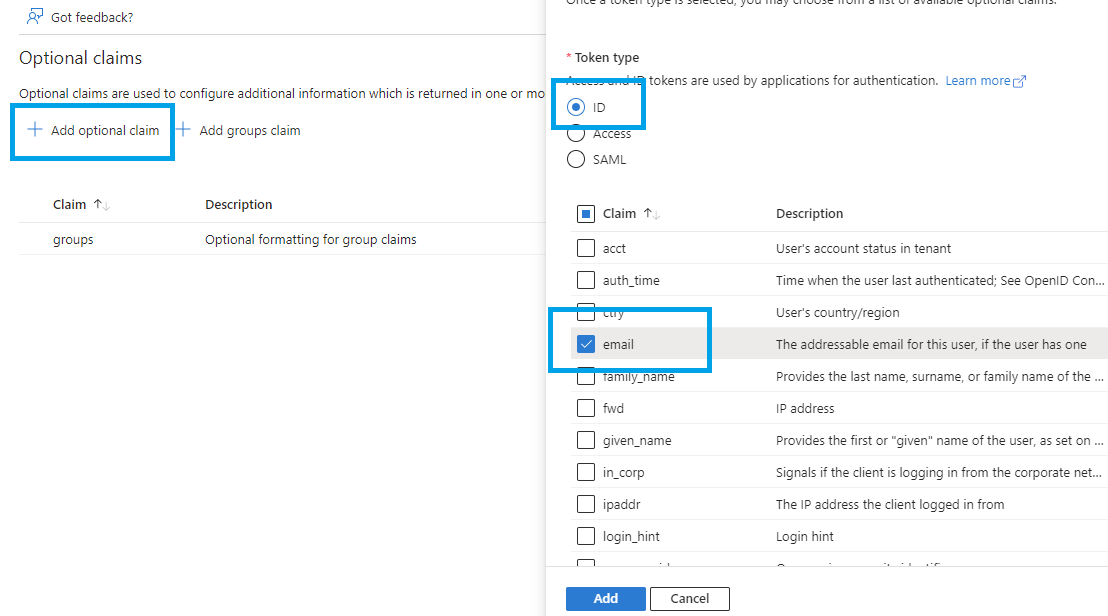The image shows a computer screen with two different pages displayed side by side. The page on the left features a user interface with a small person icon followed by the text, "Got Feedback," prompting the user to type their input. Below this, there's a section titled "Optional Claims," which includes a brief description that states these claims are used to configure additional information. Some of the descriptive text is cut off, indicating there is more content below the visible portion. A blue button labeled "Add Optional Claim or Add Group Claims" is also visible, along with additional information related to claims.

The right page, which is partially obscured at the top with the upper part of the text cut off, appears to have an overlay effect. The key elements on this page include sections titled "Token Type" and a list format that allows users to click on various claim options. Particular emphasis is given to two boxes labeled "ID" and "Email," both of which are prominently highlighted in blue, suggesting they are important focal points within the interface.